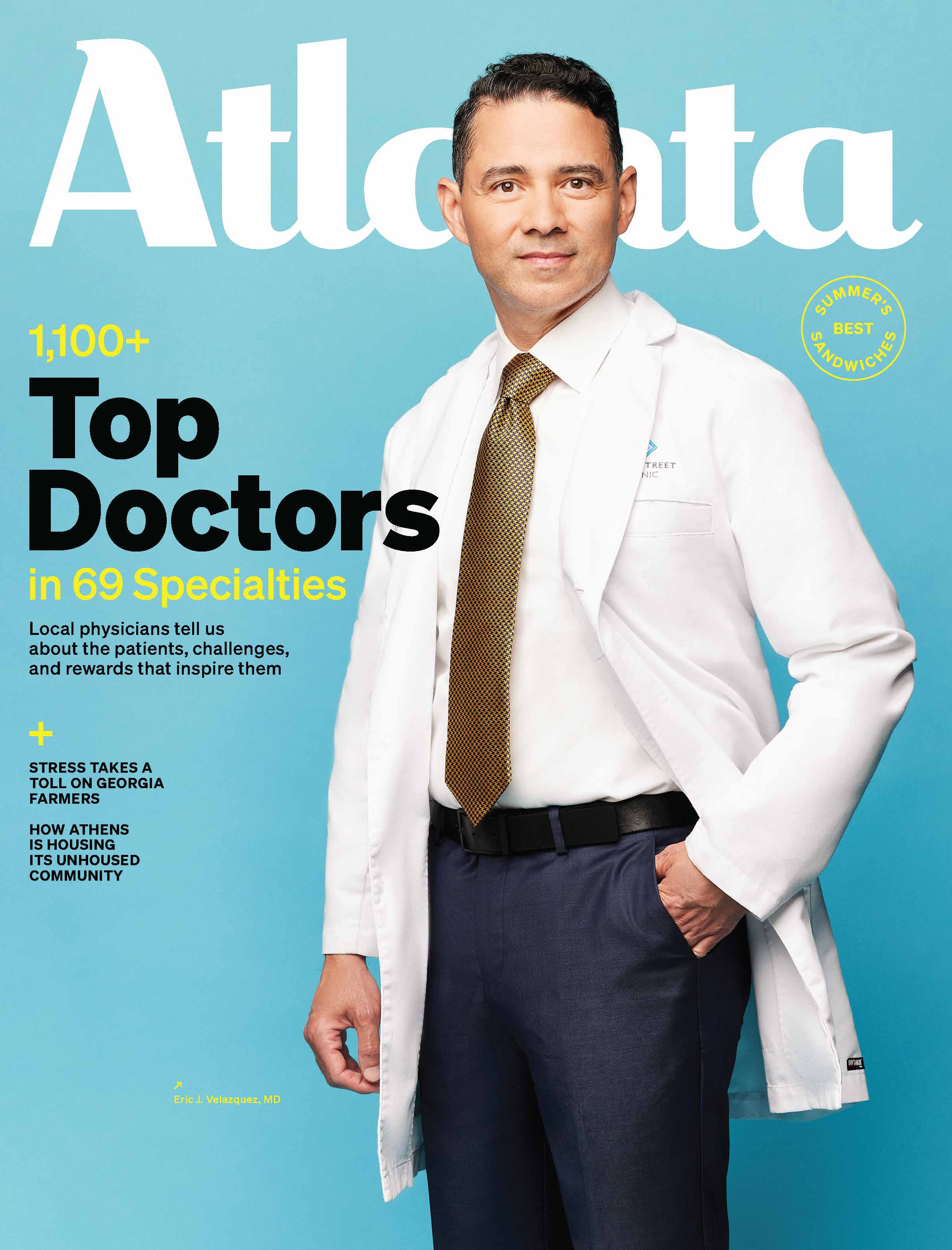The cover of the "Atlanta" magazine, presumably based in Atlanta, Georgia, features a striking three-quarters length photograph of a white male, who is likely a doctor, dressed in a white doctor's coat, a white undershirt, a gold dotted tie, steel gray pants, and a black belt. This male model has his left hand partially tucked into the pocket of his coat. The background of the cover is a light turquoise blue, and the magazine's title "Atlanta" is displayed in white text at the top. 

Dominating the design is the bold headline in varying fonts and colors: “1,100+ Top Doctors in 69 Specialties,” with "1,100+" and "in 69 specialties" highlighted in yellow, and "Top Doctors" in larger, black font. Beneath this, a subheadline reads, “Local physicians tell us about the patients, challenges, and rewards that inspire them.” Additional featured stories include discussions on how stress impacts Georgia farmers, how Athens is addressing homelessness in 179 communities, and a piece titled "Summer’s Best Sandwiches." At the bottom of the cover, there is a mention of someone with the title "Velasquez MD," although the full name is not completely legible.